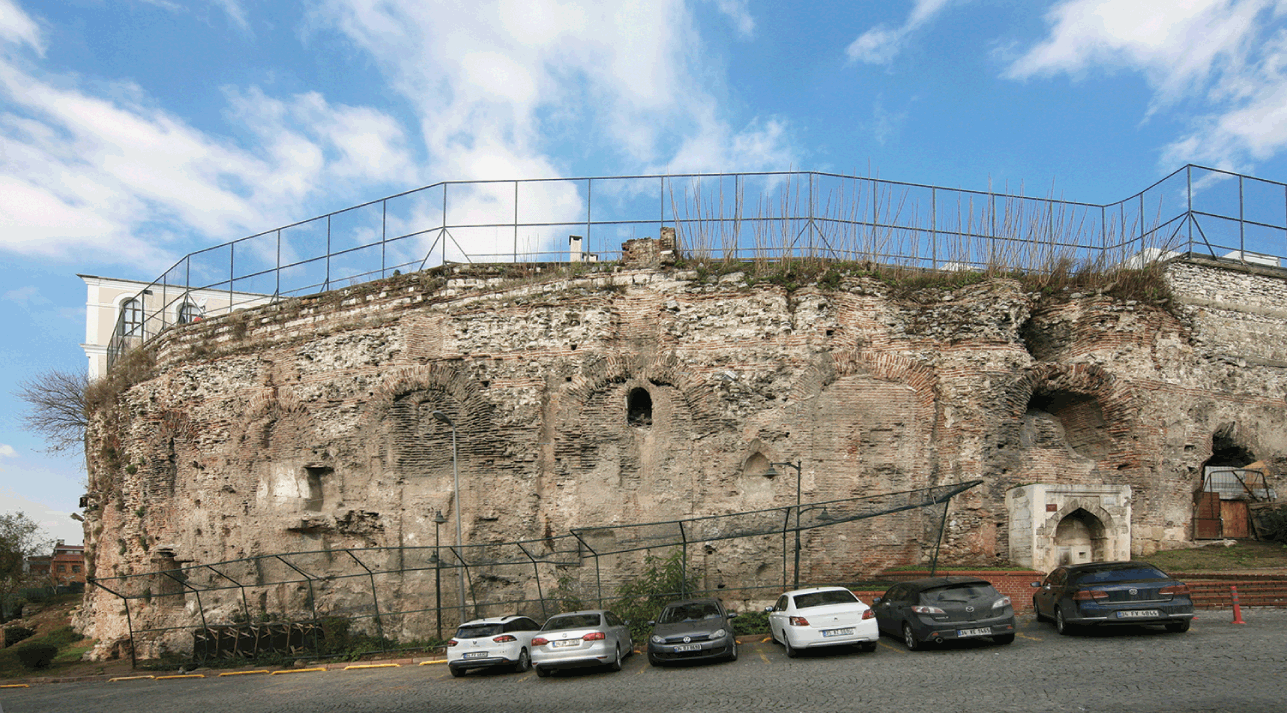In this outdoor image, we see a historical site that appears to be an old fortification or possibly a centuries-old structure carved into the side of a cliff or mountain. The center of the image is dominated by a large stone wall with worn openings that suggest it once had windows or entrances, now inaccessible and weathered by time. At the base of this structure, on the right-hand side, there is an apparent entranceway marked by white stones.

Surrounding the fortification are multiple fences; a chain-link fence runs along the top of the wall, likely to prevent people from accidentally falling off, and another darker fence separates the park area, including the parking lot, from the historical structure itself. A smaller brick wall, approximately two feet high, is also present.

In the foreground, a parking lot is visible with six cars, including three white cars, two gray cars, and one that may be gray or green. Identifying the specific models is difficult, though some might be Toyotas. Some cars are parked head-in and others backed into the spaces, demarcated by yellow parking blocks. An orange traffic cone adds a splash of color to the otherwise neutral palette of grays, whites, and brick orange hues. The sky above is partly cloudy, with patches of blue sky and white clouds, contributing to the bright daylight setting.

This location is likely a tourist destination, preserved for visitors to experience a piece of history.